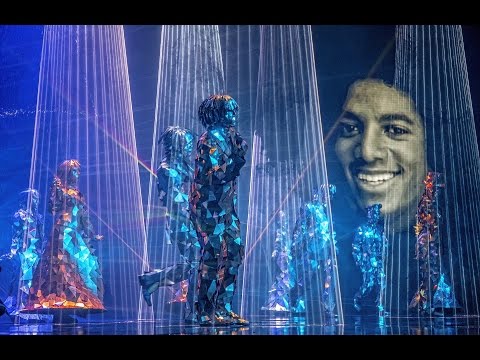The image captures a vibrant stage performance featuring polygonal humanoid figures with a metallic and reflective finish, predominantly in silvery blue hues with some elements showing orange and reddish tones, possibly due to lighting effects. These geometric performers, resembling either crystalline or robotic structures, appear to be engaged in a dance, with light beams cascading down from the ceiling and creating dynamic reflections on the floor. The stage is framed in black, enhancing the brightness of the light beams. In the background, the monochromatic portrait of a younger Michael Jackson is visible, lending an iconic touch to the scene. There is a mix of outfits among the figures: a prominent figure in the forefront dons a silver outfit with black trim, another in the background wears a silver dress, and one distinct character stands out in a reflective red dress. The overall effect is a captivating blend of light, color, and geometric artistry on stage.